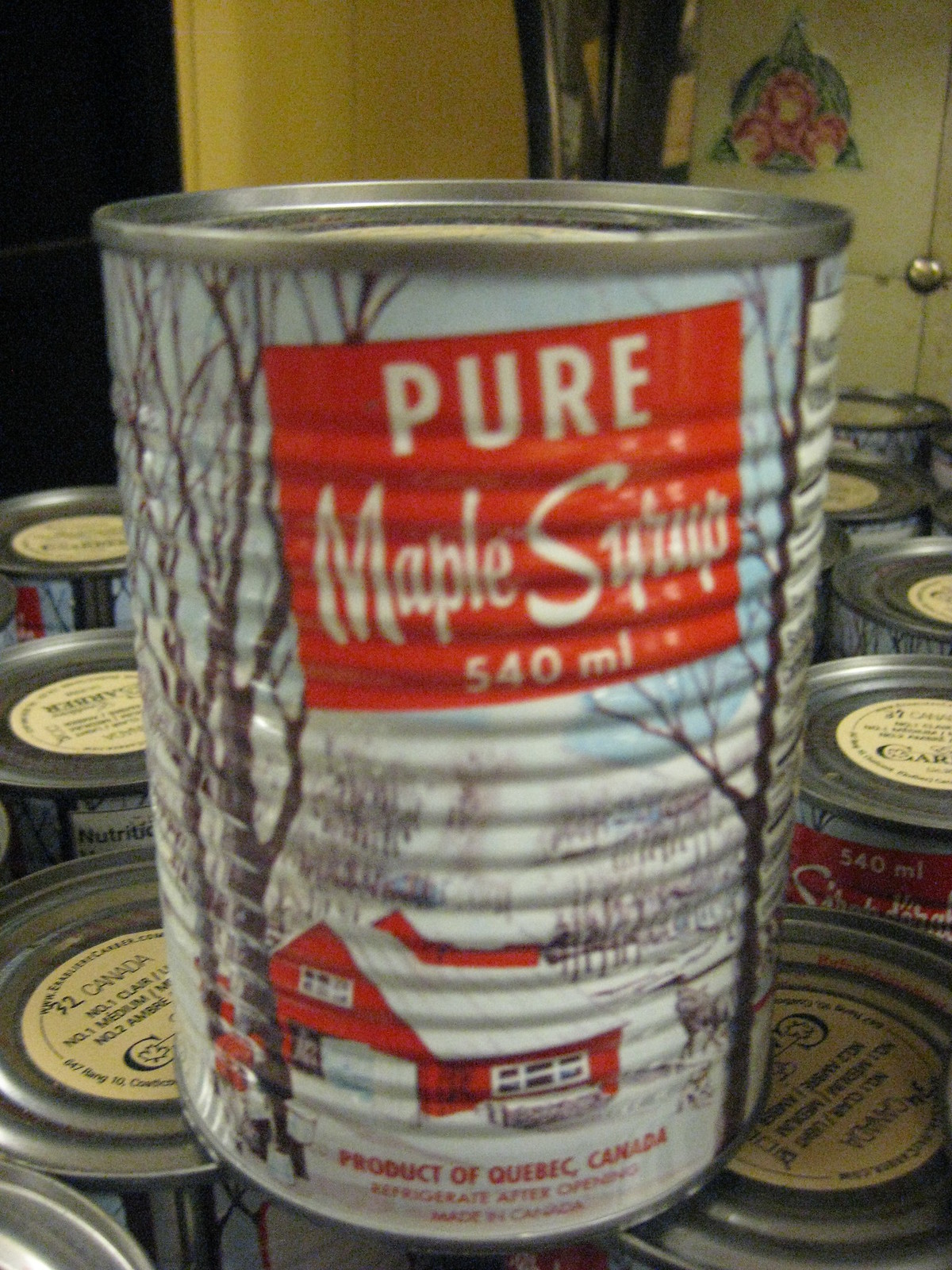This photograph, taken in an interior setting with a mustard yellow wall and dark green cloth stripe, prominently features a tin can of pure maple syrup, specifically 540 milliliters. The can, made of tin or aluminum and with a corrugated surface, has a vibrant label seemingly painted on, depicting a detailed winter scene. The label has a white and blue background, the blue representing the sky with clouds and the white symbolizing snow. It also showcases a red, wooden barn or cottage with white trim on the windows and roof, covered in snow. Surrounding the cottage are several leafless tree trunks and snowy ground. The red rectangular area at the top of the can states "pure maple syrup 540 ml" in white text. Below, additional text reads "Product of Quebec, Canada" and advises to "Refrigerate after opening," confirming it was "Made in Canada." The can is stacked on several identical cans, whose lids are visible, with a yellow sticker on top detailing more information such as "Canada number one medium" and a checked tick box. The background of the image includes a dark brown feature, possibly a door or closet, and an upper right segment with a partially visible door adorned with a green and pink drawing and a silver handle.